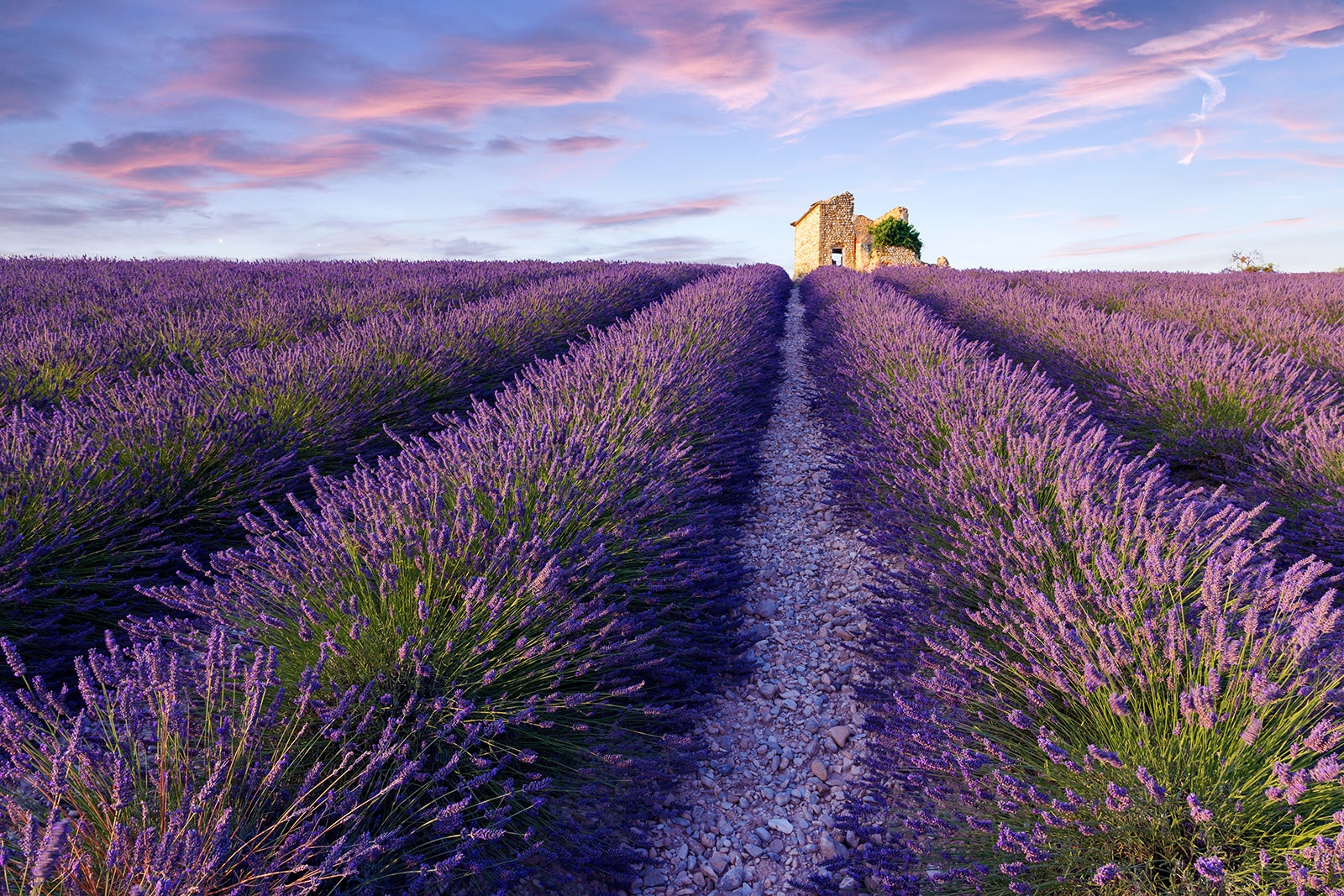In the photograph, a captivating landscape unfolds under a twilight sky, tinged with hues of purples and pinks suggesting an approaching sunset. The sky transitions from blue to soft purple and pink, with wispy and puffy clouds enhancing the serene atmosphere. The ground below is dominated by meticulously arranged rows of lavender shrubs. These shrubs, each about one and a half to two feet tall and around three feet wide, present an array of vibrant purple blossoms at the ends of their green stalks, creating a dense, colorful tapestry. Running through the rows is a gravel pathway, tinted slightly pinkish-purple, inviting onlookers to traverse the fragrant field. Off in the distance, slightly to the right of center, stands a crumbling yellow stone building, evocative of archaic ruins, possibly centuries old. A large tree rises from within the ruins, adding to the historic and timeless feel of the scene. The combination of the purple sky and the blooming lavender creates an enchanting and picturesque moment, blending nature's beauty with a hint of historical mystique.